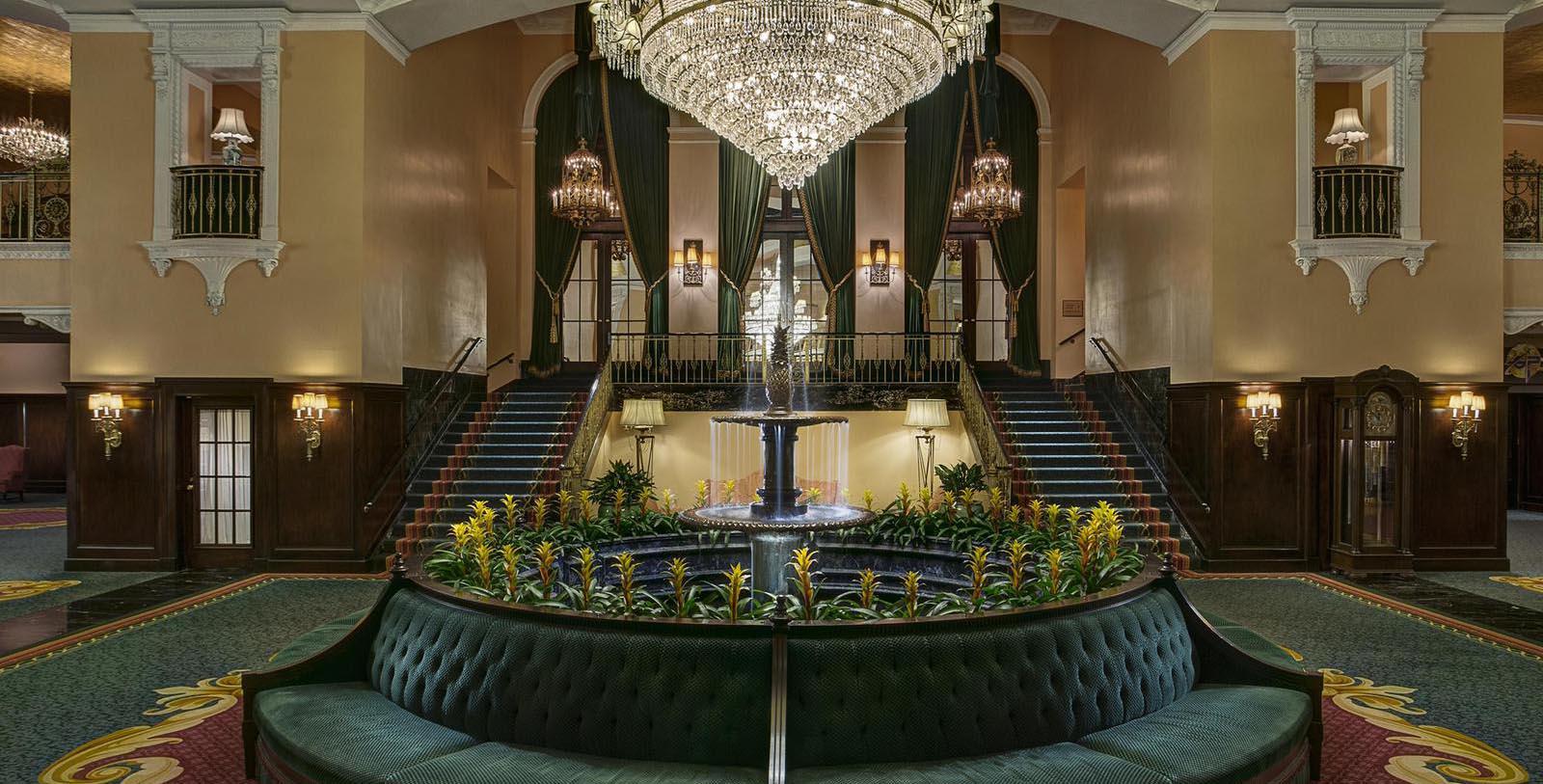The interior appears to be a luxurious lobby, possibly of a high-end hotel or an opera house. The space is defined by its opulent detailing, featuring a large, eye-catching crystal chandelier forming a conical shape that descends from the ceiling, surrounded by smaller crystal chandeliers. The ambiance is enhanced by the warm glow from the chandeliers, yellow lamps on the walls, and illuminated sconces.

Central to the room is a round seating area with green velvet chairs arranged in a circular fashion around a large fountain. The fountain is adorned with yellow flowers and lush green foliage, creating a serene focal point. This central seating arrangement allows guests to sit with their backs to the fountain, providing a relaxing environment.

The flooring showcases an elaborate carpet, featuring gold scallops with maroon accents, which adds to the grandeur of the space. This carpet extends to two grand staircases on either side of the fountain, both carpeted to match. These staircases lead up to a balcony and additional entries with green curtains and large windows in the background. The staircases are accompanied by white-trimmed, tan walls and decorative pillars, giving the structure an elegant symmetry.

Additional notable details include small verandas with lamps, a matching carpet on the stairs leading up to other rooms, and a grandfather clock positioned near the right staircase. The overall decor reflects a sophisticated and harmonious blend of detailed design elements, making for an exquisite and visually captivating lobby.